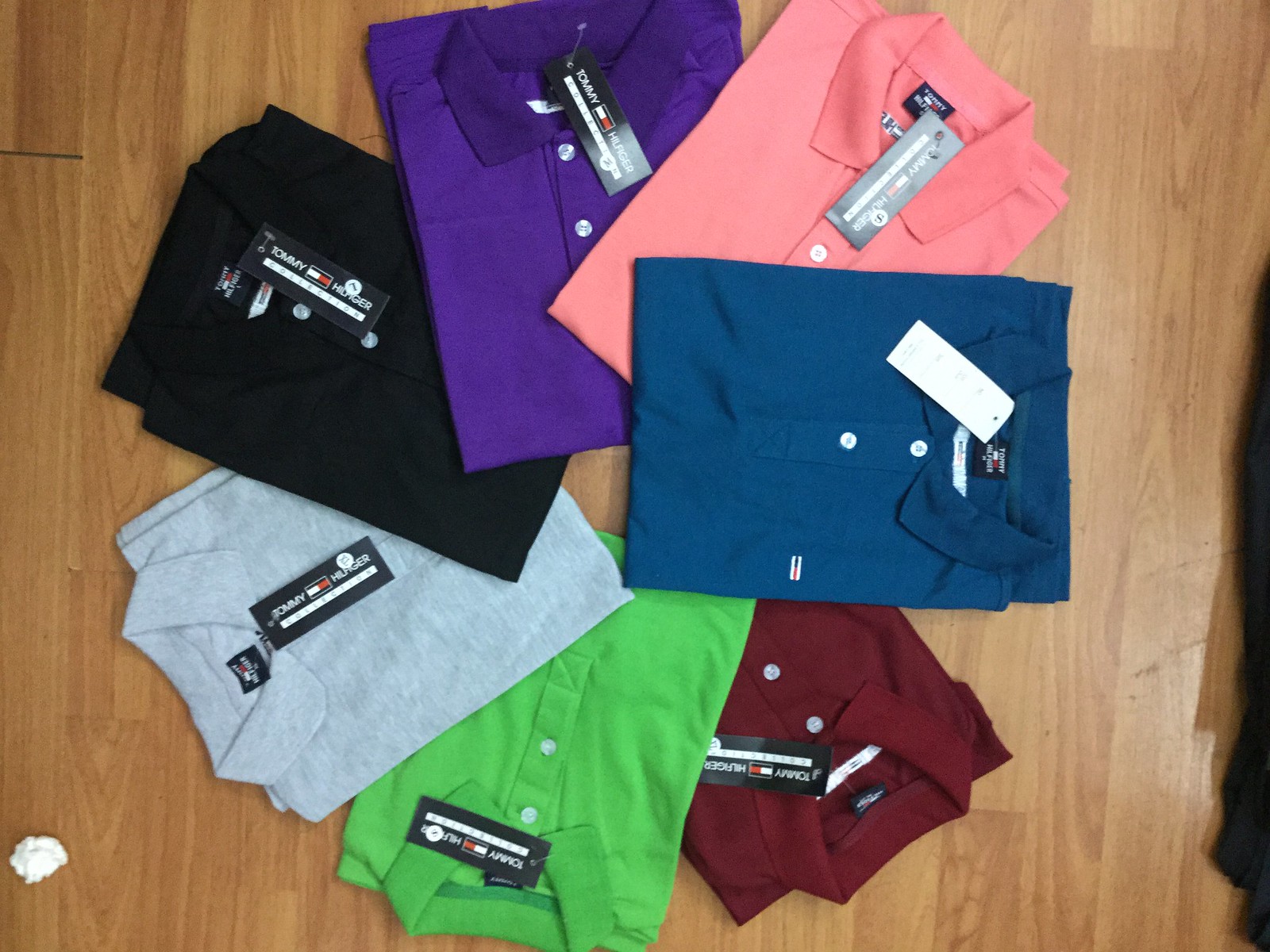In this top-down photograph, a collection of Tommy Hilfiger polo shirts are meticulously arranged in an overlapping spiral pattern on a hardwood floor. Each shirt, still brand new with tags attached, is folded neatly in a typical store display fashion, with sleeves tucked in to form square or rectangular shapes. Starting from the top and moving clockwise, the shirts are displayed in the following colors: deep purple, pink, navy blue, burgundy, green, gray, and black. Each polo shirt features white buttons and a collar, indicative of classic tennis or polo shirt styles. In the bottom left-hand corner of the image, a crumpled piece of tissue is visible, while a small, indistinct black garment peeks into the frame on the right.